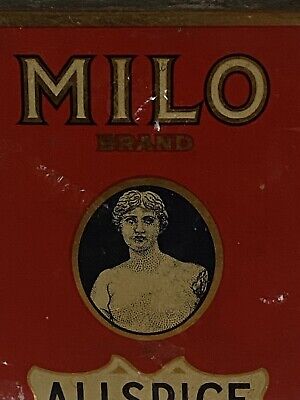The image appears to feature a vintage label, possibly from an old-fashioned can of spice or a cigarette brand. The background is a deep red or burgundy color, bordered by a dark frame which suggests it might be a small poster or a label on a can. 

At the top of the label, the word "Milo" is prominently displayed, followed by some partially obscured text that might say "brand." In the center, there is an illustration within an oval or circular frame depicting a Greek statue, identifiable by its classical styling and missing arms, visible only up to the upper chest. Below the statue, the text "All Spice" is somewhat legible but partly cut off, further hinting at the label being an old can of allspice. The label exhibits signs of aging, including scuff marks and stains.

Overall, it presents an antiquated appearance, suggesting that it might be a vintage product label displayed on a website.